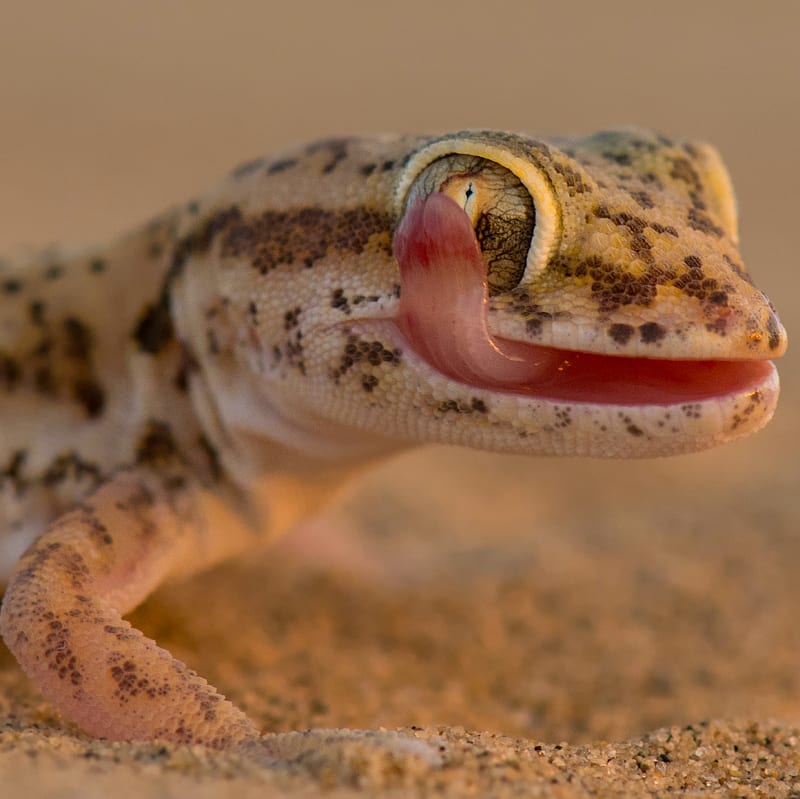This close-up, professional nature photograph captures a gecko blending seamlessly into its sandy environment. The gecko's textured scales are predominantly tan, accented with dark brown and yellow spots and lines, camouflaging perfectly with the beige-tan sand it stands on. Its underbelly features contrasting white scales. Dominating the frame, the gecko's head is oriented to the right, with a vividly pink tongue extended to lick its large, intricate eye, which is a mix of tan, dark brown, yellow, and white with a glint of sunlight reflecting off it. The gecko's mouth is slightly open, revealing its pink interior. In the blurred background, the sandy environment continues, enhancing the gecko's camouflage. Two tiny pink nostrils are visible on the top of its nose, and its right front leg is partially seen pressing into the sand. The detailed granules of sand are especially clear in the foreground, adding to the image's intricate and immersive quality.